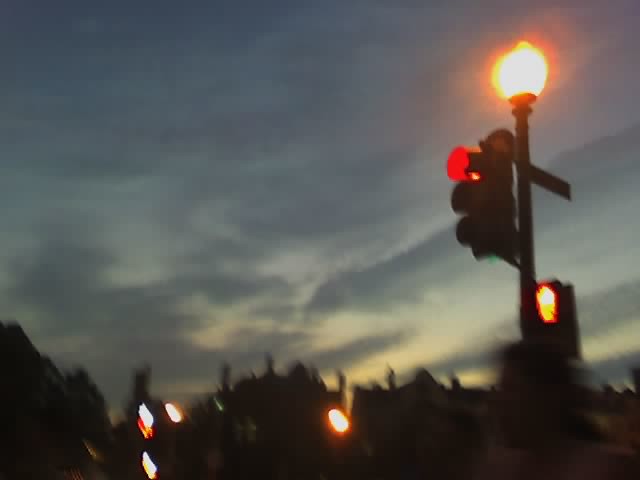The image is a pixelated and blurry digital photograph, possibly an enlarged version of an original, capturing a city skyline at sunset. The scene showcases the silhouette of various buildings against a darkening sky. To the right of the image, a street lamp glows brightly, its post running parallel to the image's right edge. A traffic light displaying a red signal is positioned to the left of the street lamp. The bottom of the image is dotted with three or four indistinct blobs of light, likely emanating from building windows or streetlights. The sky transitions from a dark gray at the top to a smoky yellow near the horizon, emphasizing the fading light of dusk.